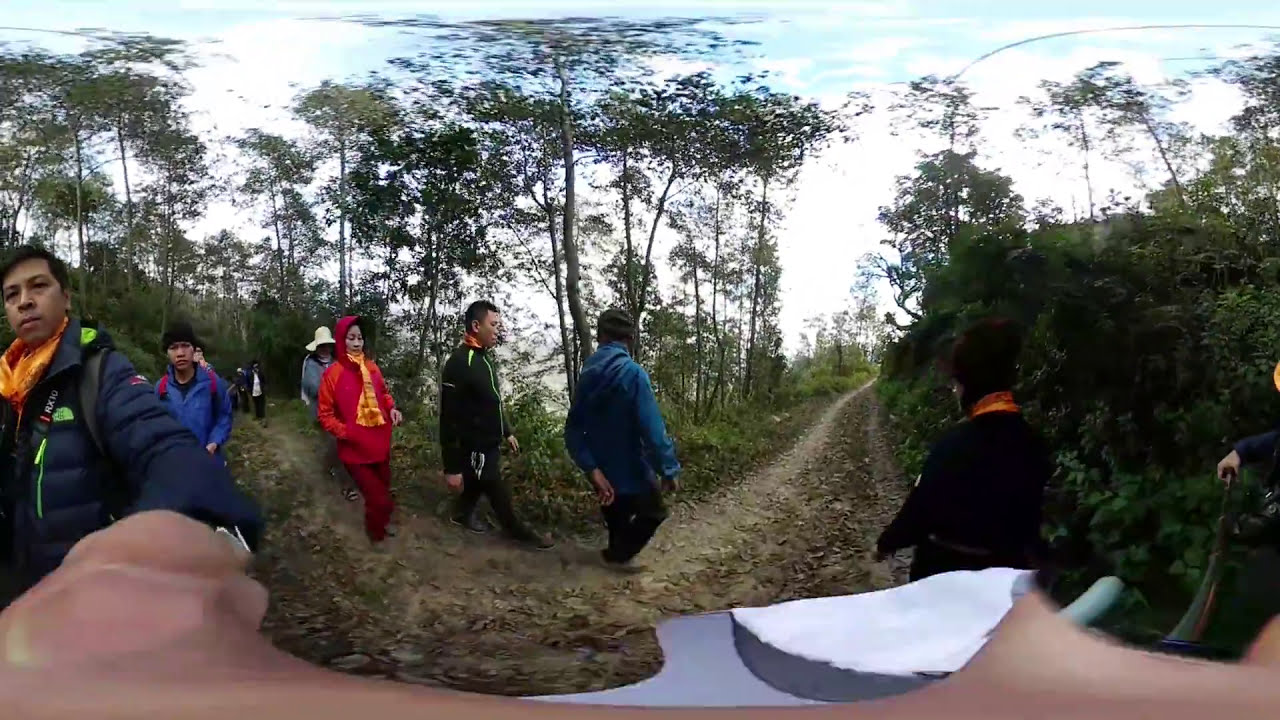The image depicts a group of hikers, all appearing to be of Asian descent, traversing a green, wooded trail under overcast skies. The photo, captured using a 360-degree camera, shows a man in a black puffer jacket with an orange scarf prominently on the left side of the image, his arm and the camera pole visible on the right side due to the extreme fisheye effect. In the background, a boy in a light blue jacket and a woman dressed in red with a yellow scarf are visible, along with two men walking ahead of them. The dirt path is light brown and adorned with rocks, bordered by lush green foliage and trees. This midday outdoor setting is vibrant with various colors including blue, red, green, and gray, emphasizing the lively, albeit distorted, scene of a communal hike.